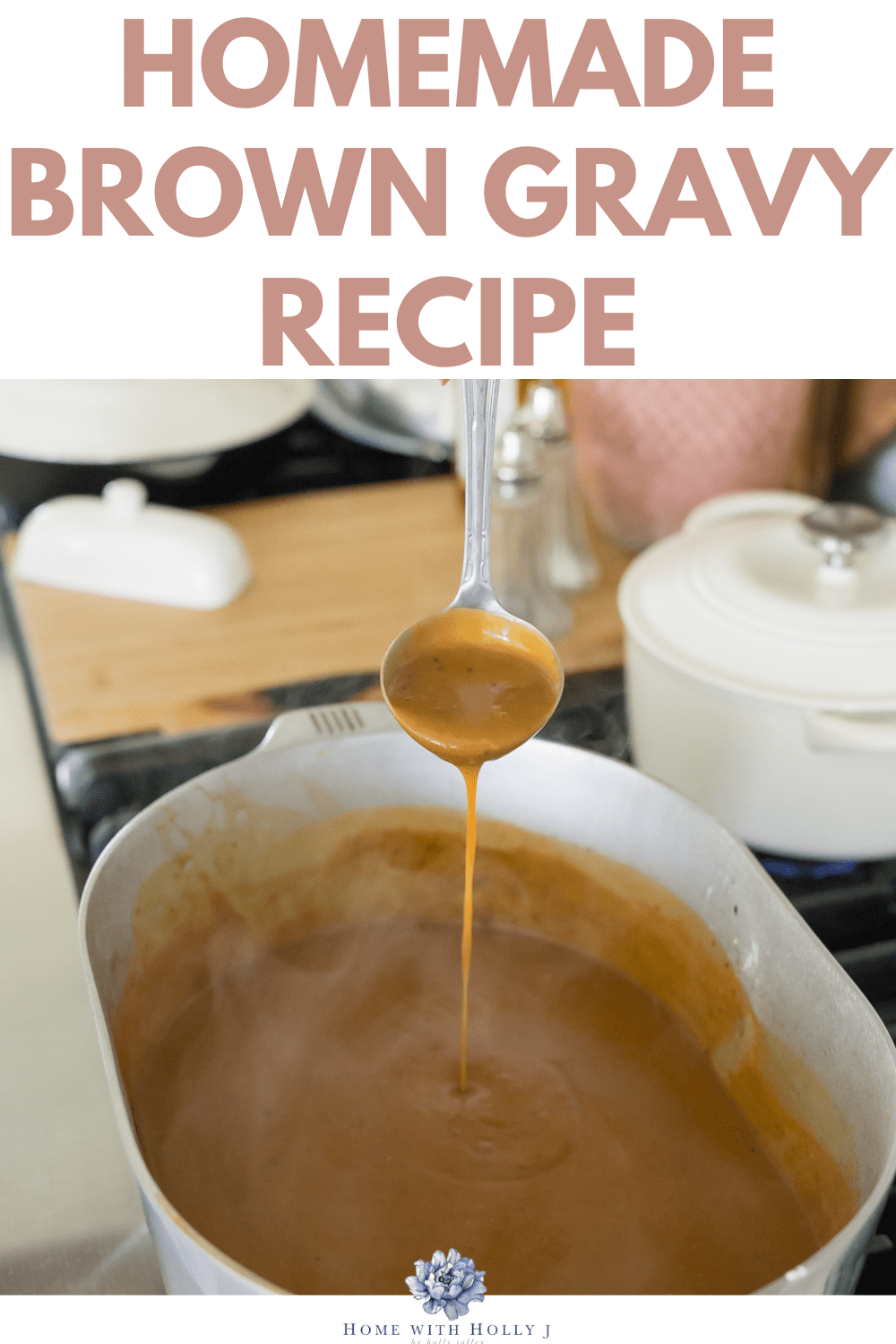The image captures a page that might be from a recipe book or a screenshot of a video, prominently featuring a white oblong casserole dish filled with light brown gravy. A ladle extends from the dish, letting the gravy drip back into the vessel in a thin stream. The backdrop consists of a vaguely discernible wooden surface, along with a salt and pepper shaker, and to the right, a white pot with a lid. Behind the white pot, there's a blurry pinkish object. Above the casserole dish, text in light brown font against a white background reads "Homemade Brown Gravy Recipe." At the bottom of the image is an illustration of a lavender flower, and underneath it, in blue font, it says "Home with Holly J."